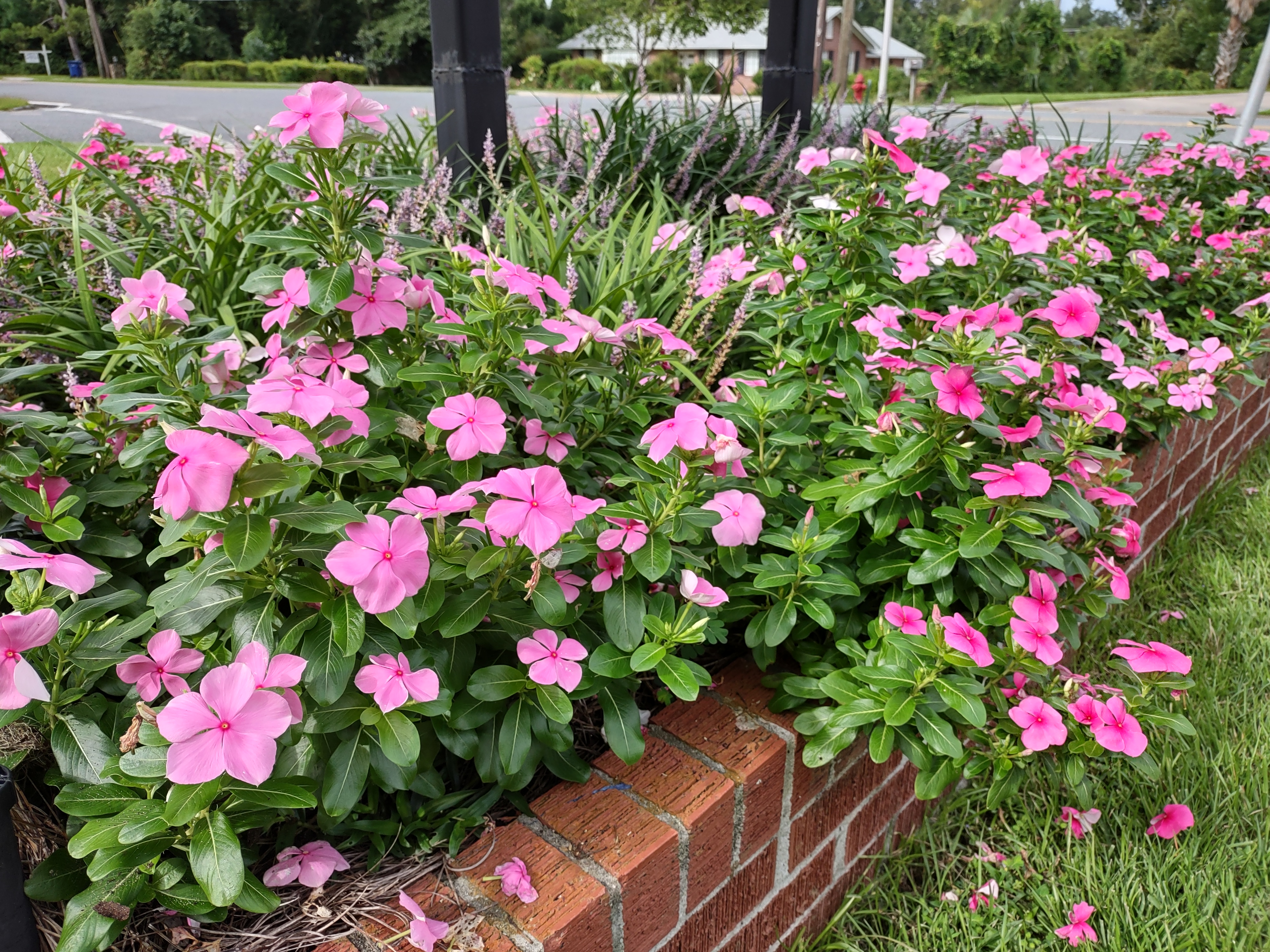The image features an outdoor scene capturing a vibrant flower garden encased in a brownish brick structure. The brick enclosure is made up of perpendicular and horizontally laid bricks, creating a distinct border around the garden. Inside, plentiful waxy green leaves support a variety of pink flowers. These flowers, which include different shades ranging from light to dark pink, exhibit five to six petals each. Some flowers have tiny pinkish-purple centers, while others feature larger, more pronounced centers of a similar color. Additionally, a white sign and a blue trash can are visible near one corner of the flower bed, implying the garden might be situated near a street intersection or a shopping center. In the background, across the road, stands a brick house with black shutters and a light gray roof, accompanied by trees and bushes, completing the picturesque setting.